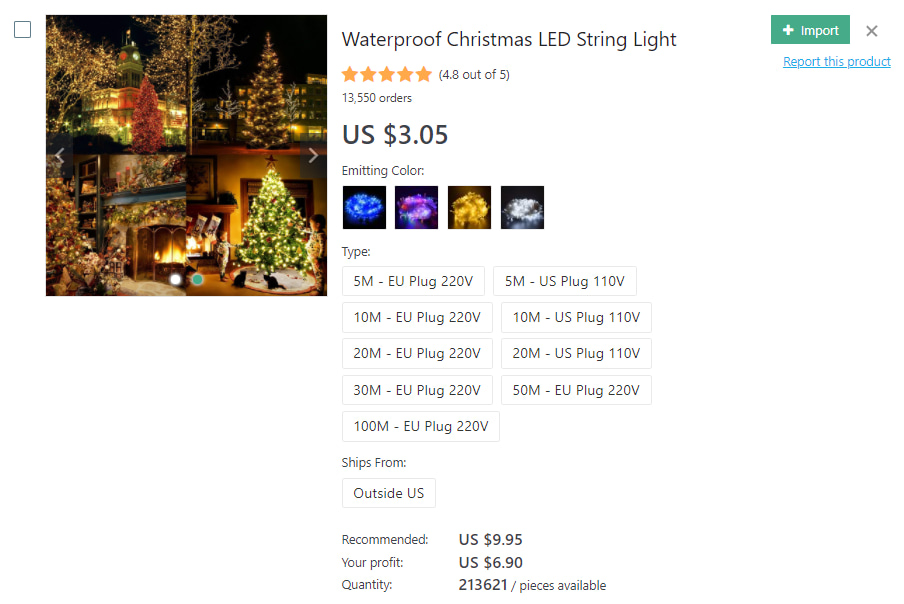This screenshot from a website showcases a product listing for waterproof Christmas LED string lights. The main section of the image is divided into four interconnected panels, each depicting different festive scenes. 

1. The top-left panel captures an outdoor Christmas setting featuring a tall building adorned with a red Christmas tree and several leafless, illuminated trees.
2. The top-right panel displays a nighttime scene with a prominent tall Christmas tree, smaller trees in the background, and a building set against a black sky.
3. The bottom-left panel offers an interior view of a cozy living room, complete with a decorated Christmas tree, lit fireplace, mantle, and bookshelves.
4. The bottom-right panel highlights a fully decorated Christmas tree with two boys, two cats, and a fireplace adorned with stockings.

Flanking the central panels are left and right navigation arrows, allowing users to scroll through additional images. 

The product information below the images reads: "Waterproof Christmas LED String Light," with a rating of 4.8 stars out of 5 from 13,550 orders. The price is listed as US $3.05, available in several colors including blue, purple, yellow, and white. It mentions that the item ships from outside the US and recommends a price of US $9.95, suggesting a profit margin of $6.90. The available quantity is 213,621 pieces.